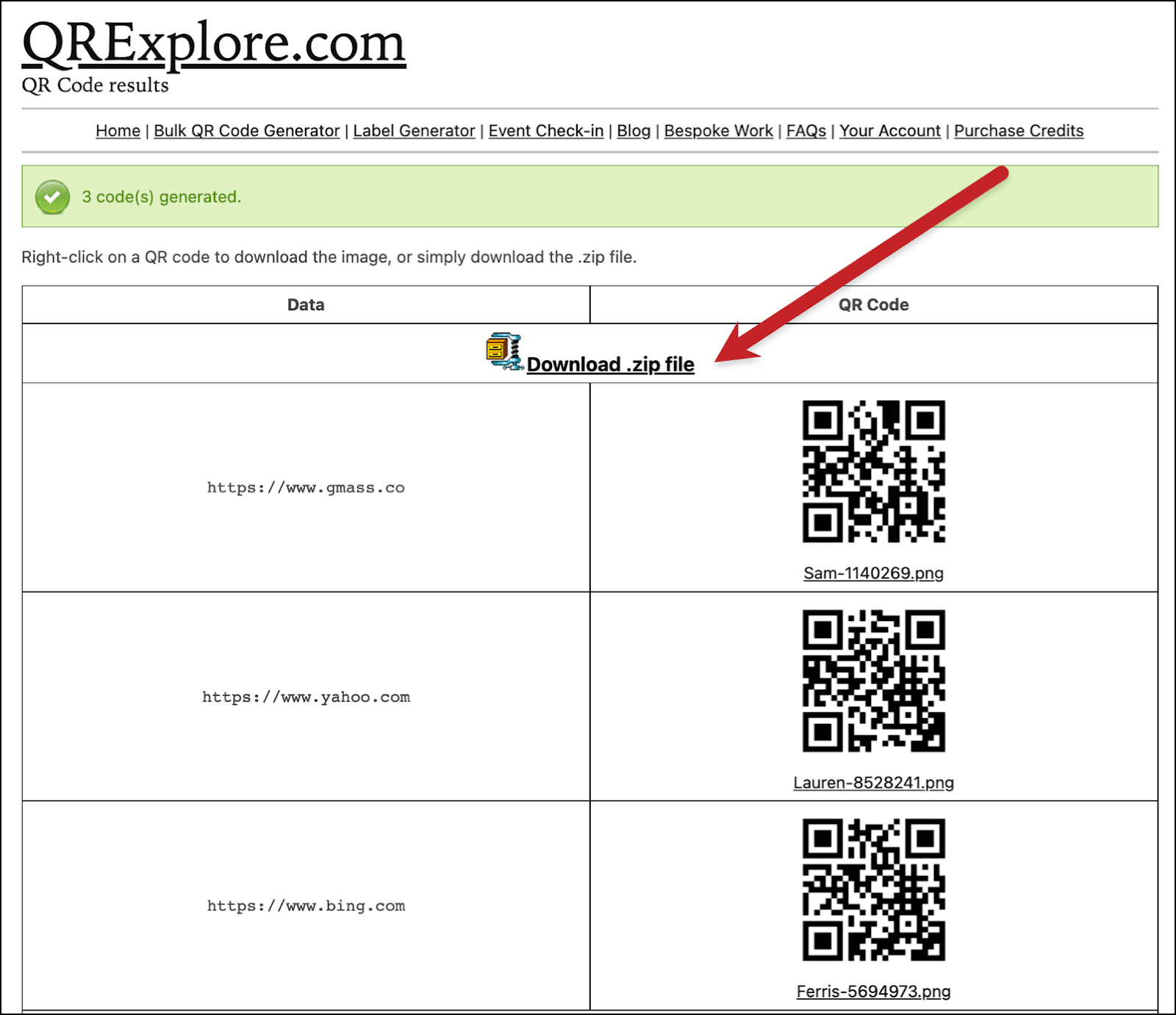This is an image from qrexplorer.com. The background is white with a very thin black outline encompassing the outside of the square. In the top left corner, the website name, "qrexplorer.com," is prominently displayed in bold text, underlined by a black line. Below that, a smaller black text reads "QR code results," separated by a light gray horizontal line. 

Directly underneath this line is a horizontal menu with links in this order: "Home," "Bulk QR Code Generator," "Label Generator," "Event Check-In," "Blog," "Bespoke Work," "FAQs," "Your Account," and "Purchase Credits."

Further down, a long light green rectangle stretches across the width of the square, containing a darker green circle with a white check mark on the left side. To its right, green text announces, "Three codes generated."

Continuing down the image, black text on the white background instructs, "Right-click on a QR code to download the image or simply download the zip file." Below this instruction are two long white rectangles in black text labeled "Data" and "QR Code."

Subsequently, there is an option to "Download zip file," highlighted by a long red arrow pointing downward toward it.

At the bottom part of the image, two vertically stacked rows of rectangles are shown. The left column features web addresses: "https://www.gmass.co" in the top rectangle, "https://www.yahoo.com" in the middle rectangle, and "https://www.bing.com" in the bottom rectangle. Correspondingly, the right column displays their QR codes.